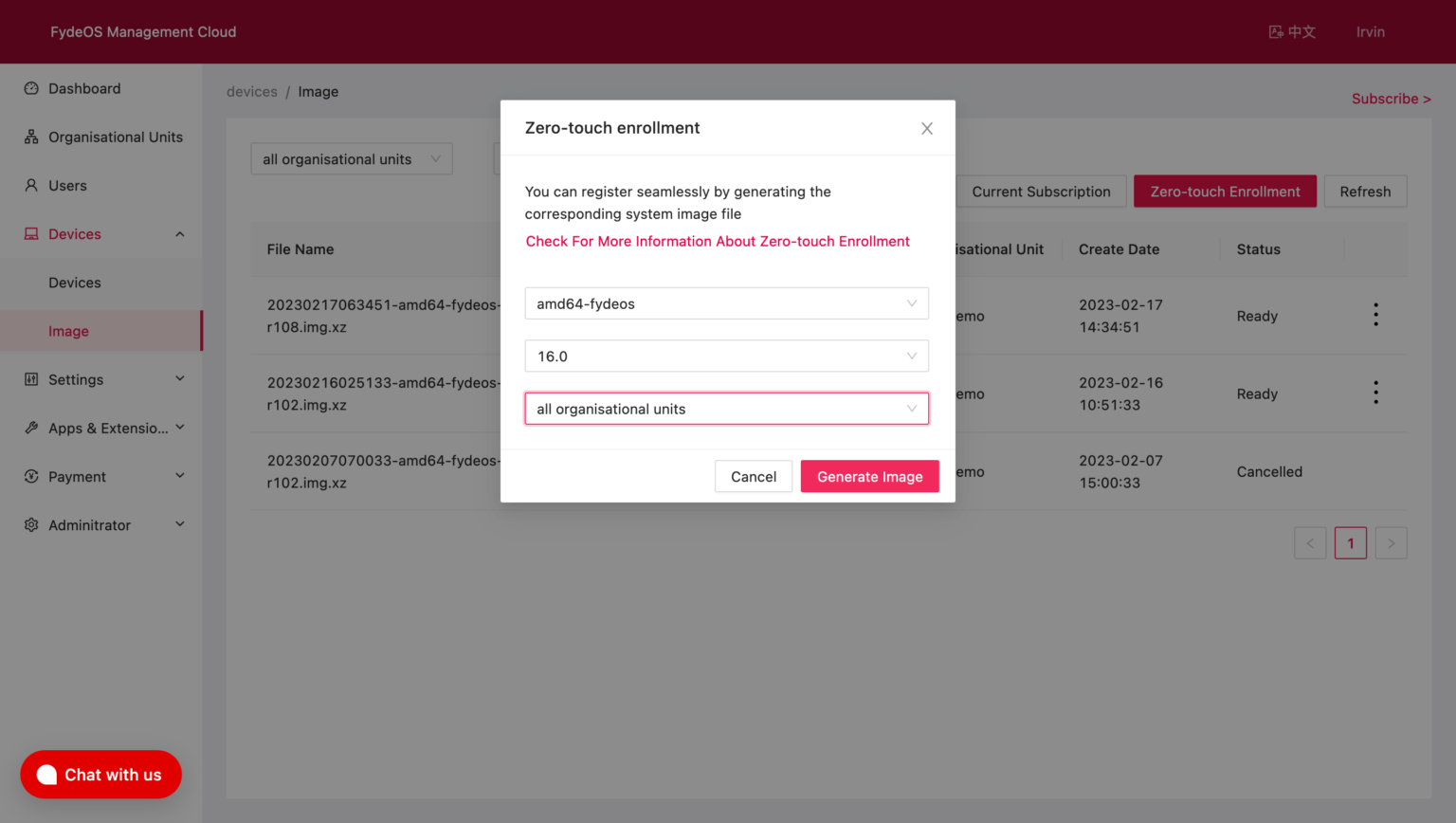This image is a detailed screenshot of a user interface for managing system image files, specifically designed for zero-touch enrollment. The layout is predominantly horizontal, with various elements organized in a clear manner. 

At the center of the screen is a prominent white rectangular box. Behind this white box, the background features a gray screenshot page. The page itself begins with a smaller white box containing both black and red text that reads: "Zero-touch enrollment. You can register seamlessly by generating the corresponding system image file. Check for more information about zero-touch enrollment."

Directly beneath this instructional text and white box is another content area labeled "AMD 64 FYDE OS." Below this section, there is a drop-down menu set to version "16.0."

On the lower right corner of the gray page, there are two buttons: "Cancel" (in a standard color) and "Generate Image" (highlighted in red), indicating the primary action.

Further backdrop elements include, in the upper left corner, a red banner displaying the text "FYDE OS Management Cloud." In the lower left corner, there's another red box with white text that says "Chat with us," offering user support and interaction.

The interface elements are carefully arranged to facilitate seamless user interaction and efficient system image file generation.